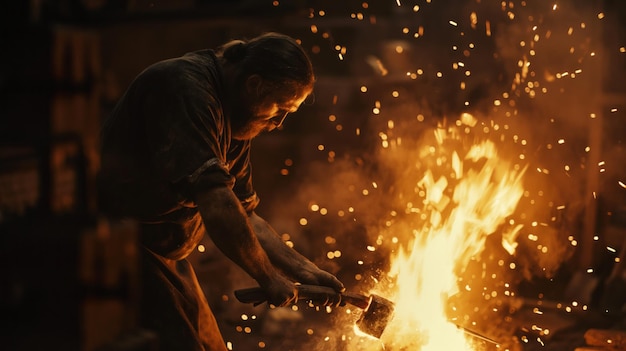The image depicts a bearded, stocky blacksmith, hunching slightly as he works in what appears to be a steel or iron-forming foundry. The man’s hair is tied back in a small ponytail, and he is dressed in a short-sleeved shirt with rolled-up sleeves and a work apron. He is seen wielding a large hammer, holding it over a bright, yellow-white flame furnace that is emitting a burst of flames and an array of sparks. The man appears to be striking a piece of molten steel within the fierce fire. The background is dark, brown, and blurry, further emphasizing the intense activity in the foreground. The vivid flames and sparks add a dynamic, almost dramatic, aura to the scene.